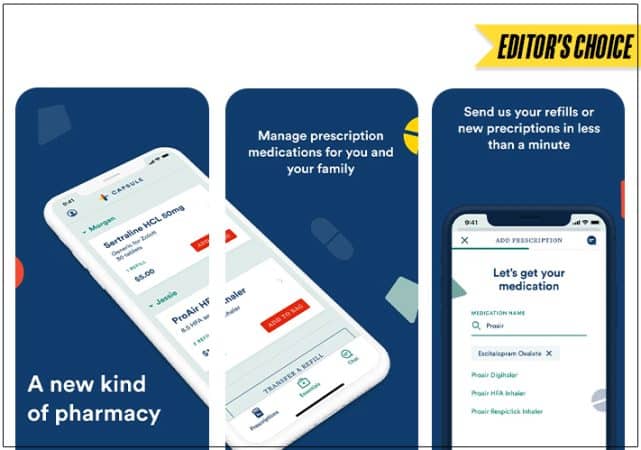This descriptive caption might fit your request:

---

This image is a promotional screenshot for a pharmacy application, displaying several notable features and design elements. The advertisement is set against a clean white background with a black-outlined, horizontal rectangular frame. In the upper right-hand corner, a yellow pennant-shaped badge with bold black letters reads "Editor's Choice," signaling a notable recommendation.

The focal point of the advertisement is a composite illustration composed of three sections, each roughly the size and shape of a smartphone screen. They feature a dark blue background with white text, creating a visually appealing contrast. Spanning the first two sections is an image of a smartphone displaying the interface of the pharmacy app, named "Capsule."

The white text prominently advertises the app's capabilities: "A new kind of pharmacy - Manage prescription medications for you and your family. Send us your refills or new prescriptions in less than a minute." Additionally, the displayed app interface exemplifies its functionality by showing prescription details, such as Sertraline HCL 50mg for $5 and a Pro-Air Inhaler. The final section features another screenshot accompanied by the text, "Let's get your medication."

---